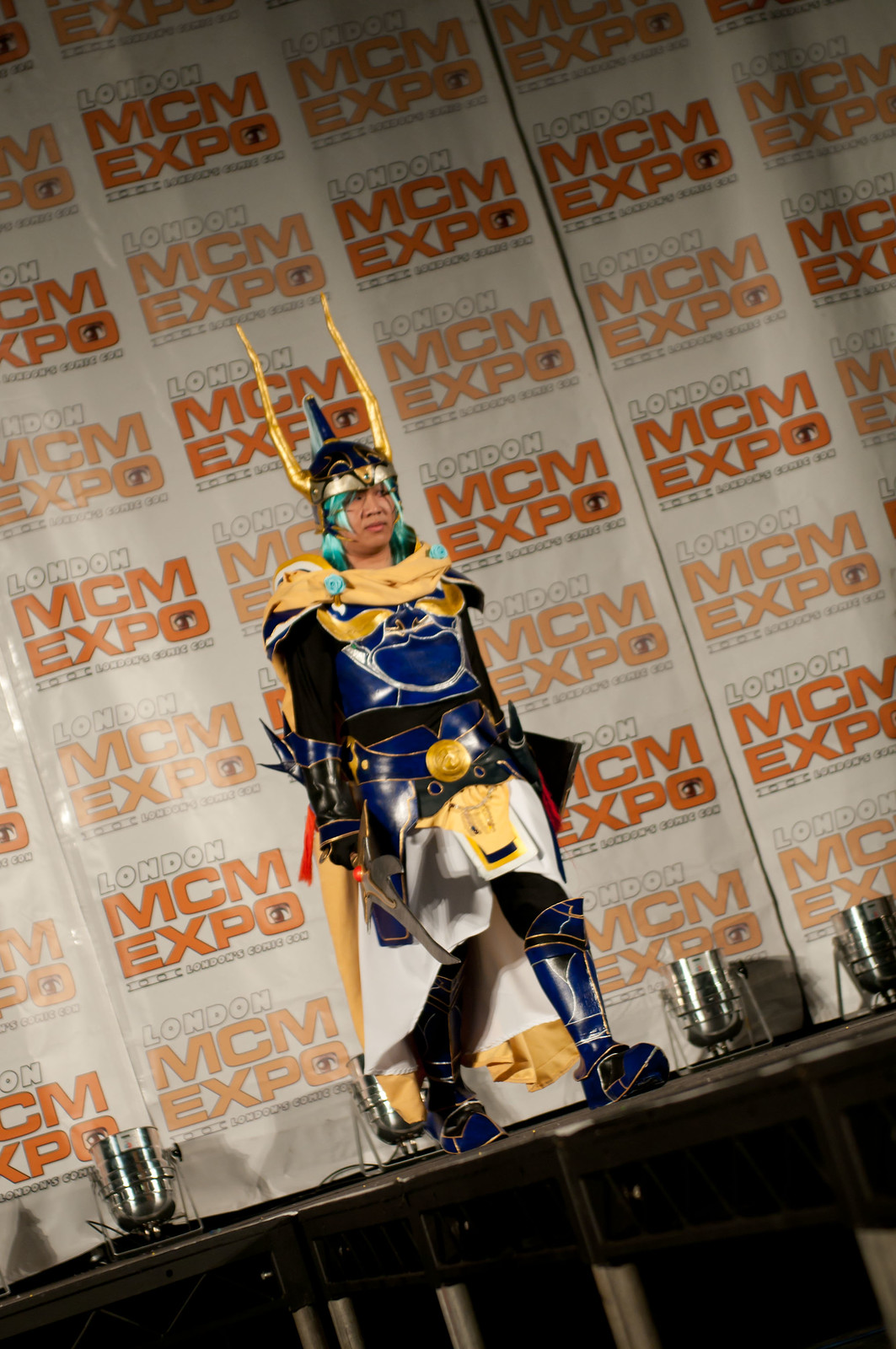A man is pictured standing on a stage, dressed in an elaborate warrior costume that appears inspired by a video game, movie, or book. The photograph is taken at an angle from the front right, with the camera tilted to the right, causing the man to appear tilted to the left in the image. Behind him, a banner with the text "MCM Expo London" is prominently displayed, repeated in a grid pattern.

The man is clad in an intricate yellow and blue ensemble. His costume features a white skirt, longer at the back than the front, accented with blue metal detailing around his waist and pelvic area, including yellow embellishments. Dominating his attire is a blue breastplate with matching shoulder pads, adorned with yellow trim for added protection. His boots and shin guards are made of the same striking blue metal. Adding to the warrior aesthetic, he wears a massive blue helmet with prominent yellow horns. He holds what appears to be a sword or similar weapon, enhancing the combat-ready look. Stage canister lights are positioned behind him, though they are not illuminated in the photograph.